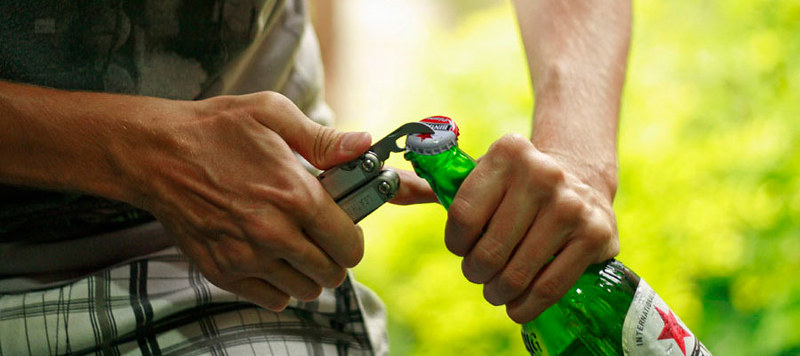A zoomed-in action image captures a Caucasian man, likely middle-aged, in the process of opening a green beer bottle with a traditional bottle opener. The man is positioned on the left side of the frame, and we can only see him from the chest to the thighs. He is wearing black and white plaid shorts and a dark-colored T-shirt, possibly gray. His veiny, lightly-haired forearms are visible, with his right hand manipulating the bottle opener and his left hand grasping the neck of the bottle. The beer bottle features a red star on its white and red cap and a matching red star on a silver label with black text, though the brand is unreadable. The blurred background, filled with green and yellow hues, suggests an outdoor setting, possibly during the summer.